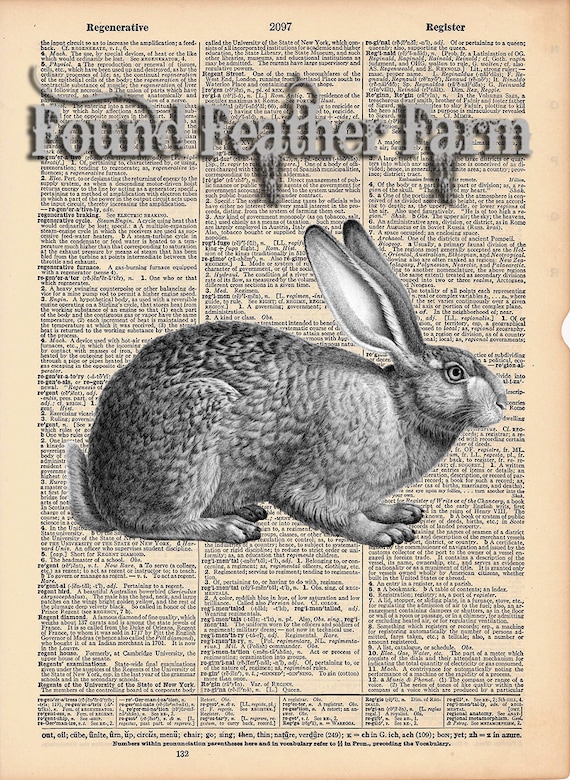The image features an intricate overlay of a vintage, newspaper-style background filled with small, unreadable columns of text, primarily in black. The background has an overall pinkish hue and includes sections with visible headings like "Regenerative," "2097," and "Register" in bold, black text. Positioned prominently atop this textured backdrop are the words "FOUND FEATHER FARM," rendered in a sophisticated gray font, with the A's in "FEATHER" and "FARM" displaying a unique melting effect. Below this, there is a detailed black and white illustration of a rabbit. This side profile of the rabbit showcases its gray-speckled fur, alert ears, and a visible eye. The rabbit is crouched on the ground, facing right, with its long ears and fluffy tail adding to its lifelike appearance.